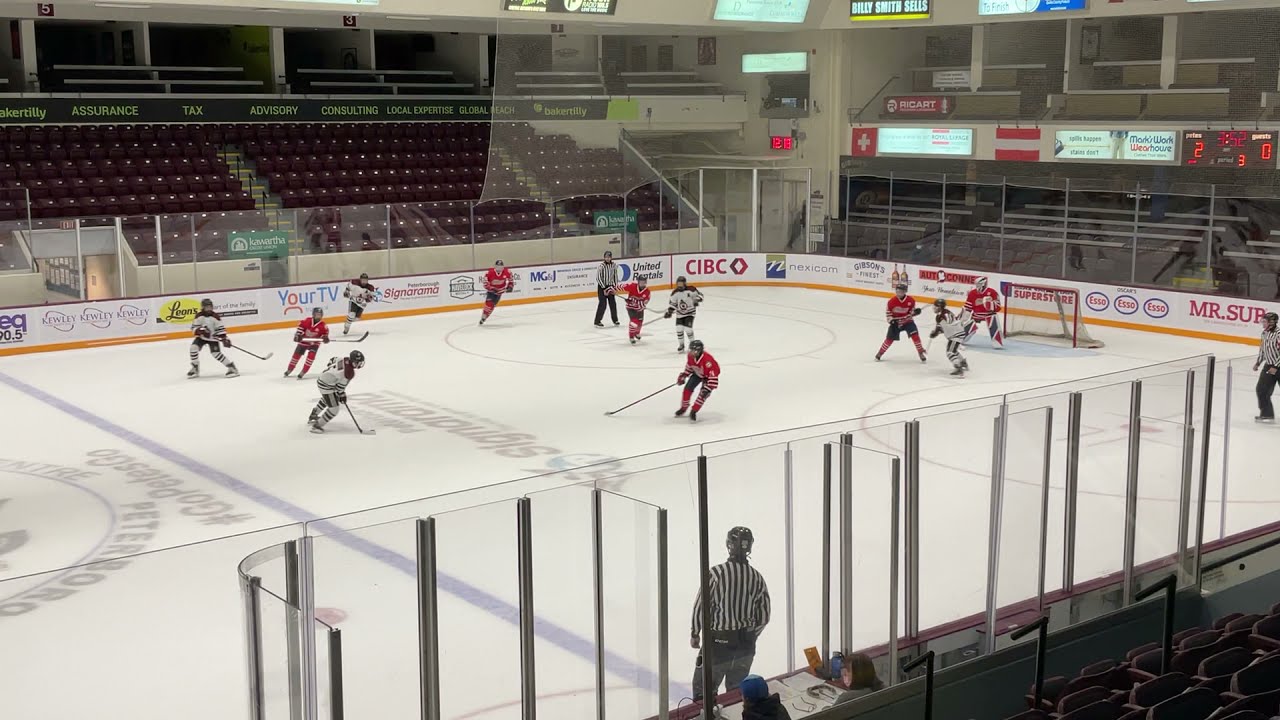In this detailed photograph of an indoor ice hockey rink, an intense ice hockey game is captured in progress. The rink is populated by ten players—five in black and white uniforms, five in red and black uniforms—and a goalie in a red uniform stationed in front of a goal net. Two referees in black and white striped shirts and dark pants are overseeing the game, one positioned closer to the action and another at a distance. The arena features empty bleacher seating, indicating there are no spectators present, which suggests that this could be a practice session or a game without an audience. The walls of the rink are adorned with various advertisements from brands such as Leon's, Your TV, Signorama, CIBC, United Rentals, Mexicom, Superstore, Esso, and Mr. Sub. An additional set of words—assurance, tax, advisory, consulting, local expertise, global reach, Baker Lilly—and a clock displaying "12:18" are visible above the seating area. A clear plastic barrier runs along the boards, protecting what would be the spectators from any flying pucks. The image also shows press or skybox stalls in the upper right corner, adding more depth to the indoor arena setting.